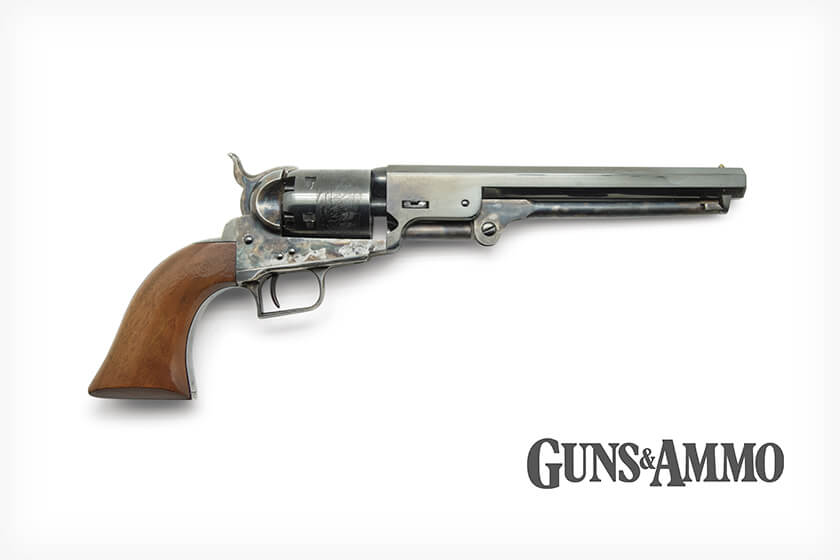This image is an advertisement featuring an old-style pistol centrally positioned against an off-white background. The gun, which prominently points to the right, has a striking silver barrel and chamber adorned with intricate, though indistinct, markings. Its handle is made of carved, dark walnut wood. Above the trigger, the gun exhibits a subtle pattern blending silver, gray, and brown hues. The safety catch appears to be engaged. In the bottom right corner of the image, the phrase "guns & ammo" is displayed in an old-style, dark gray font reminiscent of the 1950s. The overall presentation suggests a detailed product photo likely intended for a magazine.